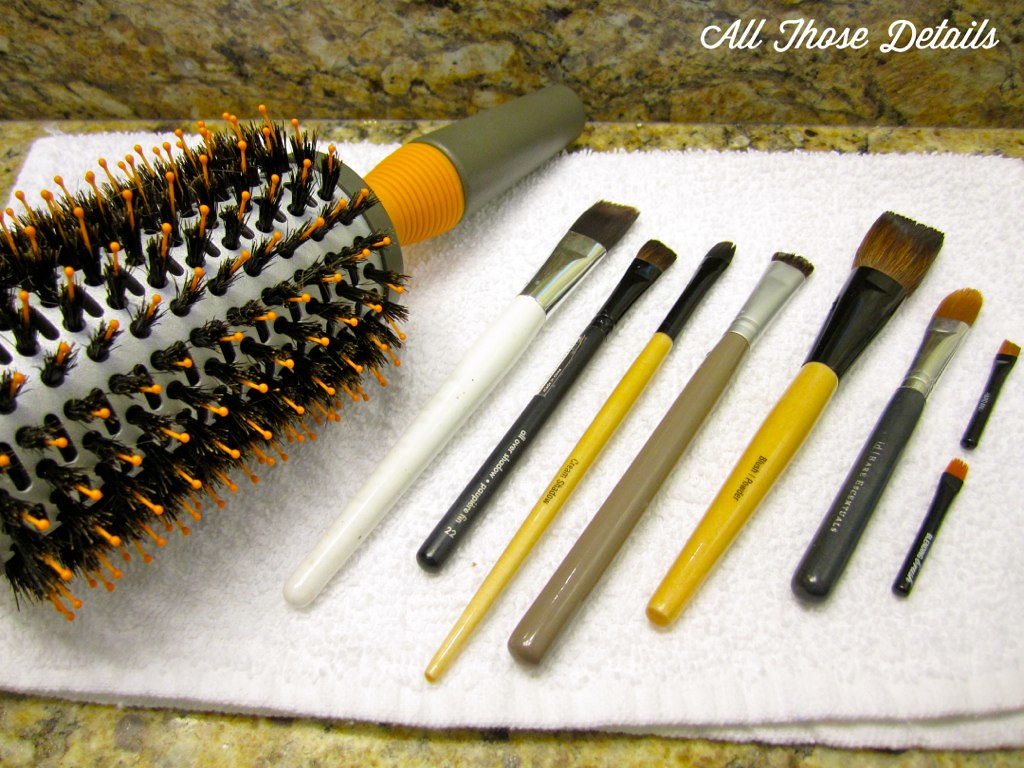In the photograph, various grooming tools are meticulously arranged on a gold and brown granite countertop. A white towel is spread out over the counter, providing a clean background for the items. Central to the arrangement is a cylindrical hairbrush, featuring a combination of black boar hair bristles and orange plastic bristles. The brush's body is silver, with the handle transitioning from gray to orange near its end. Alongside the hairbrush, there are eight makeup brushes of different lengths, widths, and bristle types, each designed for specific cosmetic applications. These brushes range from a white-handled eye brush with a silver hilt to a larger yellow-handled foundation brush with a black hilt and sharp brown bristles. Other brushes include a gray and black small brush, another yellow and black brush similar to the foundation one but smaller, and several tiny black-handled brushes with golden bristles. In the upper right corner of the image, white text reads "all those details," adding an enigmatic element to the scene.